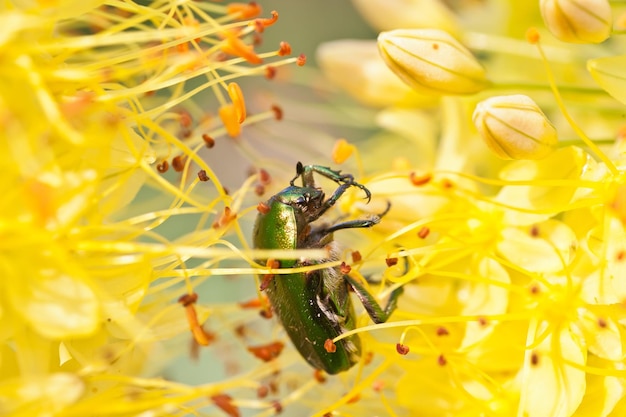In this detailed outdoor photograph, a stunning emerald green beetle with a metallic sheen and tiny black antennae is the focus, positioned prominently at the center of the image. The beetle, small yet striking, is shown climbing on bright yellow flower stamen, which extend towards it from both the left and right of the frame. These stamen consist of yellow fibers capped with orange or orangey-red tips, typical of a flower's interior. The petals themselves are yellow and some are still buds with thin green stems, ready to bloom. The background is artistically blurred, accentuating the vibrant interaction between the beetle and the flowers while highlighting a few of the closed buds with delicate lines where petals will soon emerge. The photograph captures the intricate details of the beetle, including the fine fur on its underside and the spikes on its forelegs, amid a lush but blurred green backdrop.